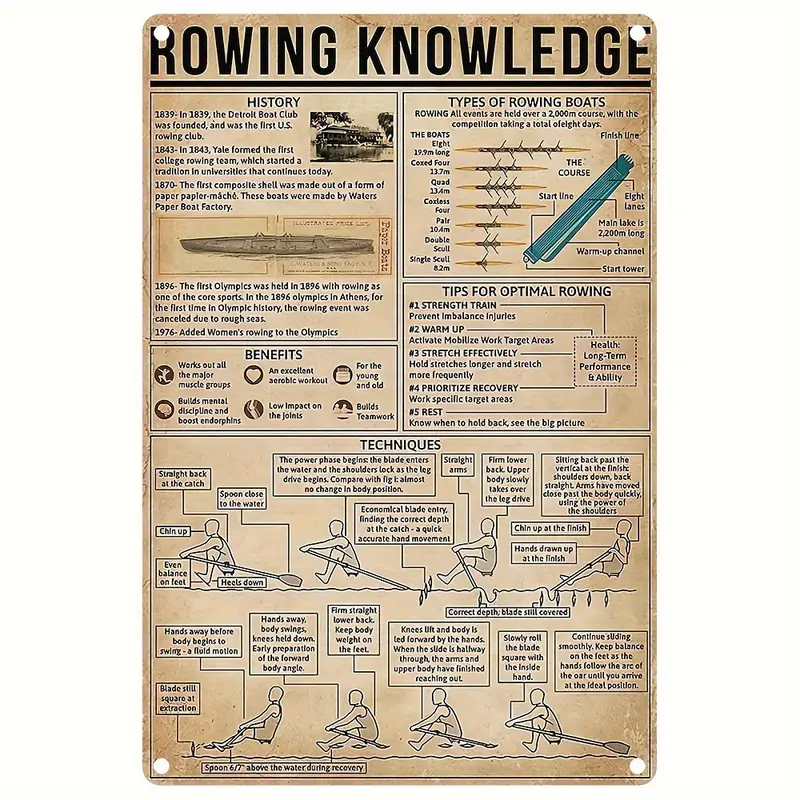The image shows an old, weathered sign that appears to have been taken off a wall, evidenced by four holes, one in each corner. The once-white sign, now turning brown with age, is titled "Rowing Knowledge" in big bold black text at the top. It's neatly organized into five sections, each with a black border around them, and is oriented in portrait format with two columns reaching about midway down the sign. The left column includes sections on the "History" of rowing (detailing events from 1939 to 1976) and the "Benefits of Rowing." The right column contains sections on "Types of Rowing Boats" and "Tips for Optimal Rowing." At the bottom, spanning the width of the sign, is a large section titled "Techniques," which features various positions for optimal rowing strokes, complete with diagrams. Most of the detailed text and diagrams within the sections are printed in blue.